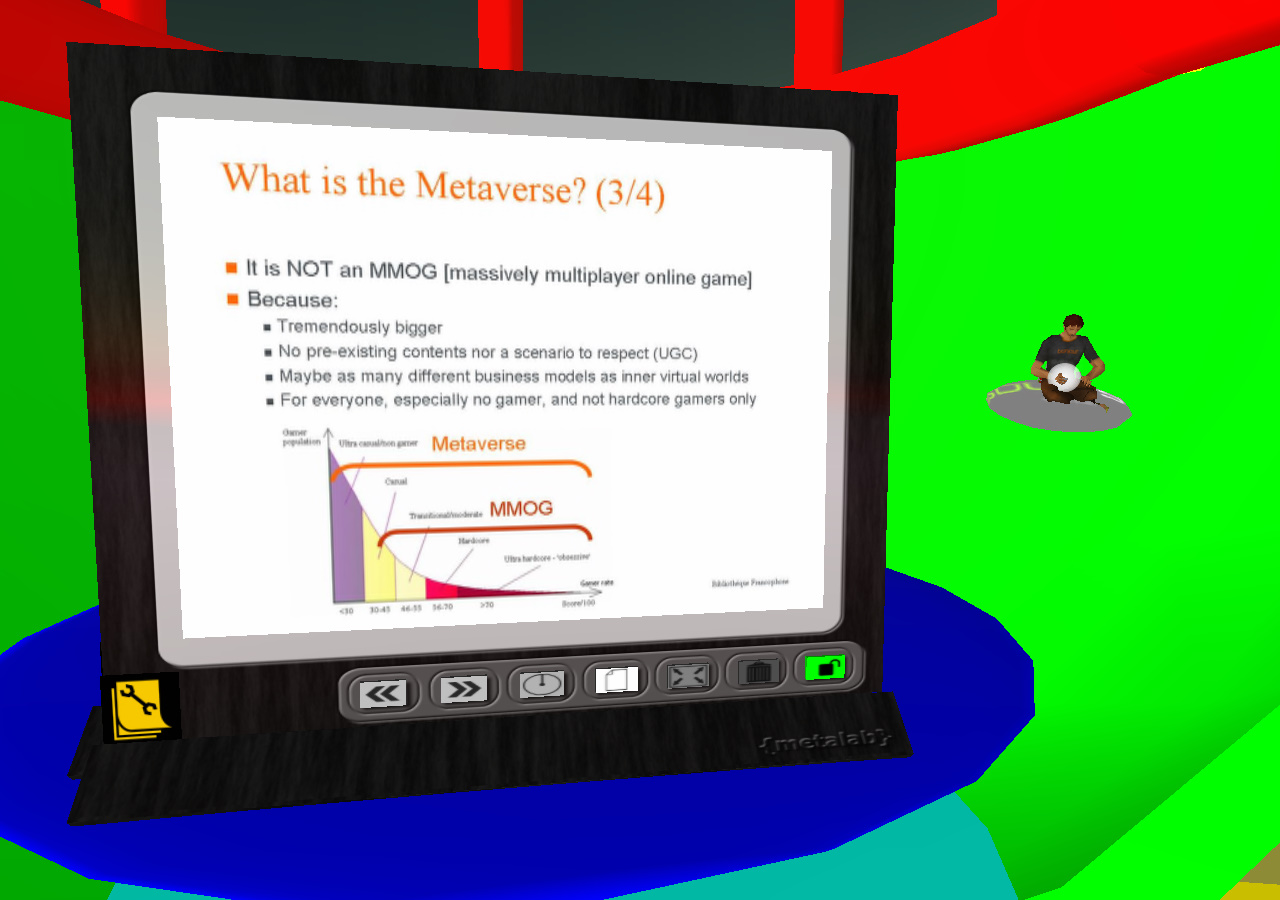This digital artwork features an animation of a computer monitor situated prominently at the center. The monitor has a black frame with identifiable buttons at the bottom for power and navigation. The display shows a white background with the title "What is the Metaverse 3/4" in orange text. Below this title, black text describes the Metaverse, distinguishing it from a massively multiplayer online game (MMOG) by indicating it is "tremendously bigger," has "no pre-existing contents nor a scenario to respect," and may support "many different business models" while being accessible to a broader audience beyond just hardcore gamers. A graph beneath this text compares the Metaverse to MMOGs, illustrating distinct aspects.

The background is detailed with vibrant colors: the right side features a curved green area where a person holding a white ball is seated on a gray circle, while the top part showcases a curved red section with circular red elements. The monitor itself rests on a flat blue circular base. This composition suggests a computer-generated setting, possibly designed for educational purposes to explain the concept of the Metaverse.